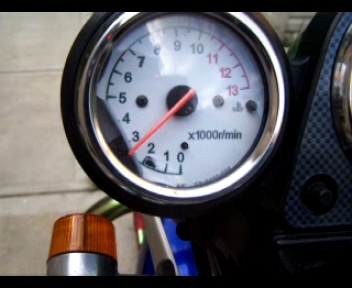Caption: 

A detailed outdoor photograph captures a motorcycle RPM gauge. The gauge, marked with "X1000R/min," displays single-digit increments from 0 to 13, and currently indicates 2.5, representing 2500 rotations per minute. To the side of the gauge, part of a carbon fiber dashboard is visible. Beneath the gauge, wooden planks are discernible, adding to the rustic atmosphere of the setting. Despite the gloomy weather, the intricacies of the gauge and surrounding details are clearly depicted.